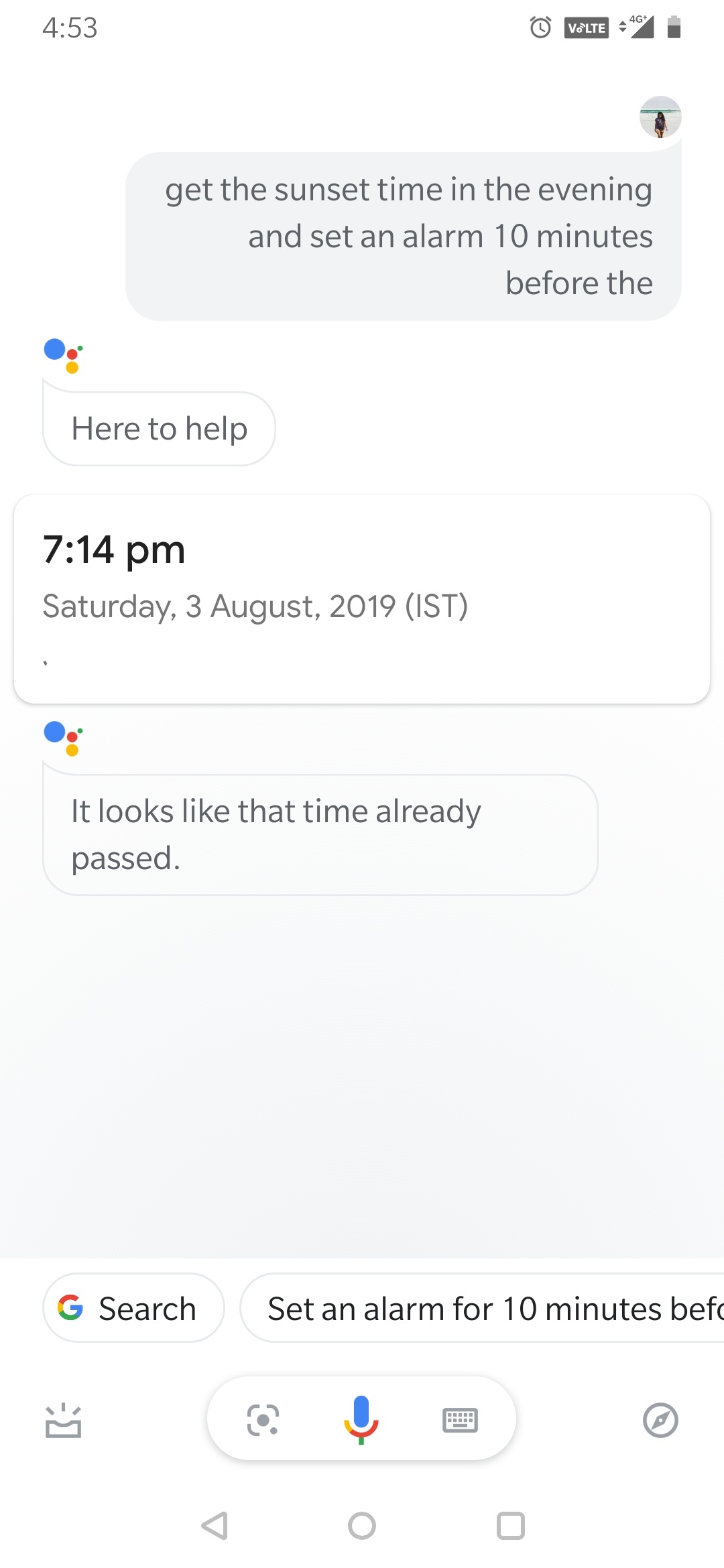A conversation displayed on a smartphone screen, likely a help or reminder app interface. The top of the screen shows status icons: "443" in gray, a gray alarm clock, a gray banner with "V-O-L-T-E," and a "4G" signal icon fully colored in, alongside a battery symbol over half full, indicated in black. 

Below these status indicators, a small, light-toned profile picture appears, depicting a girl walking on a beach with a visible sky, water, and white sand. Accompanying this, a gray banner reads, "Get the sunset time in the evening and set alarm 10 minutes before the."

Towards the left, the familiar Google dots in blue, red, and gold are present, followed by a gray "Here to help" banner. Further details include "7:14 PM" in black, and in gray, "Saturday, 3 August, 2019 (IST)." The Google dots appear again below this information with a message indicating that the mentioned time has already passed.

The remaining screen is predominantly white, with an outline of a search bar at the bottom featuring the Google logo "G" and "Search" in black text. An adjacent, cut-off icon suggests setting an alarm 10 minutes prior. In the middle of the screen, icons for voice input (a microphone in Google colors), a calendar (gray), and a camera (gray) are displayed. At the very bottom, typical smartphone navigation buttons are visible.